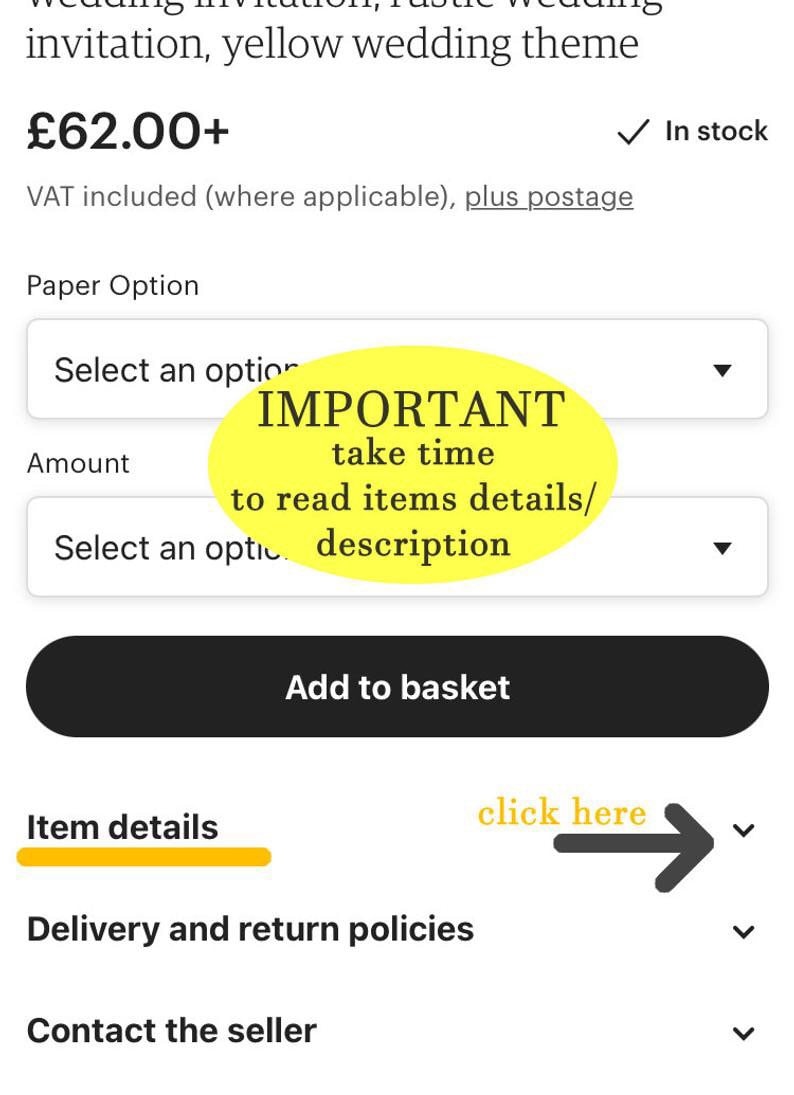This image is a screenshot of a mobile website, specifically an ordering page for wedding invitations themed in yellow. The background of the page is white, with a prominent yellow oval centrally superimposed, containing black text that emphasizes the importance of reading the item details and description.

At the top of the image, partially visible text indicates the product title: 'Invitation, Yellow Wedding Theme.' Just below this, the price is listed as £62, with a checkmark verifying the item is in stock. Additional text notes that VAT is included where applicable, with a hyperlink for further postage details indicated by underlined text saying 'plus postage.'

Beneath the pricing details are two drop-down menus: one for selecting paper options and another for choosing the quantity, both currently showing 'Select an option' as no selections have been made. Below these menus is a prominent black button with white text reading 'Add to Basket.'

Further down, there are three additional drop-down menus. The first menu, 'Item Details,' is highlighted with an underline in yellow, accompanied by a hand-drawn black arrow and the text 'Click here.' The following menus are 'Delivery and Return Policies' and 'Contact the Seller.'